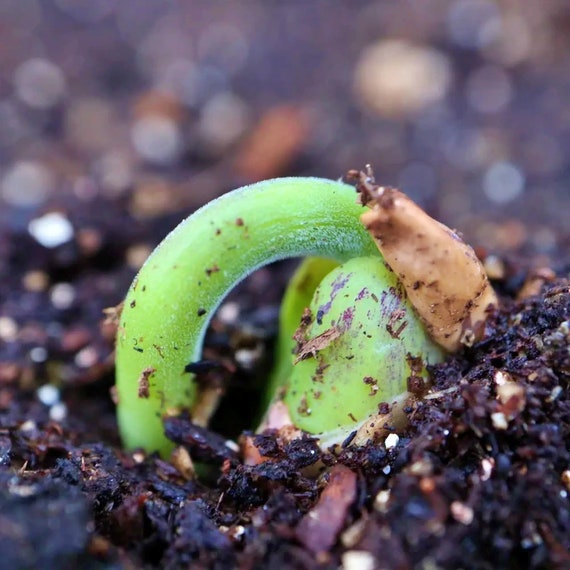This image is an ultra-close-up, professional photograph capturing the initial stage of a tiny seed sprouting. At the center of the composition, a vividly bright green sprout emerges from a partially split seed husk, which is just barely peeking above the ground. The sprout is curved, with part of it still embedded in the dark, moist soil that is peppered with white speckles, possibly fertilizer. A brown leaf can be seen adjacent to the sprout on the right side. The central focus is remarkably sharp and detailed, while the surrounding soil and possible other growths in the background are out of focus, creating a bokeh effect. The dominant colors in the image are the vibrant green of the new sprout and various shades of brown from the dirt, highlighting the freshness and vigor of new life emerging from the ground.